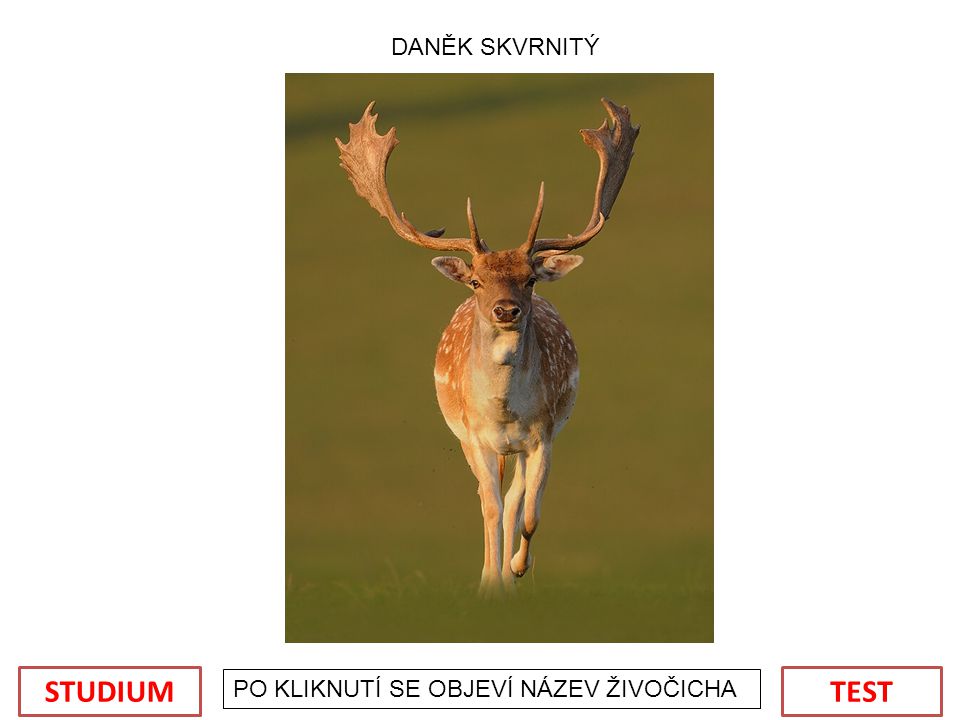The photograph prominently displays a large moose walking directly toward the viewer, providing a face-on view. The moose's fur is mostly brown with patches of white speckles, and its massive antlers, which are adorned with lighter tips, extend outward impressively, with two larger antlers parallel to each other and two smaller vertical horns on its head. Its ears stick out horizontally from its sides. The background features blurred, green hues, suggesting a grassy, outdoor setting, possibly with a hill in the background. Text in a Northern European language is positioned above the image, while more text, possibly in Polish, is found below it. Additionally, there are two red boxes at the bottom corners of the image, with the left box displaying the word "stadium" and the right one "test."